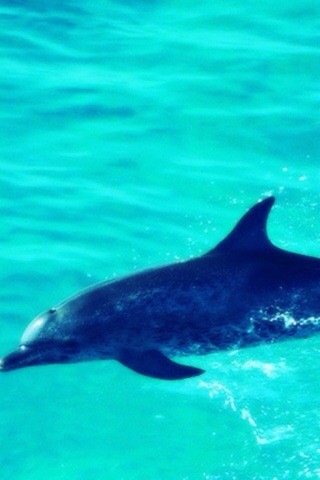This rectangular photo, reminiscent of an older camera's quality, captures a dark, dappled-gray dolphin swimming in turquoise, slightly wavy water. Three-quarters of the dolphin's body—from the tip of its nose to just past its dorsal fin—are visible, with the top third of its body breaking the water's surface. The water, tinged with darker spots and movement shadows, appears almost greenish in certain areas. The dolphin, surrounded by splash and simulating playful behavior, has a bit of glare on its forehead, indicating a bright, sunny day. The overall impression is of a dynamic and lively moment in a natural or pool-like setting.